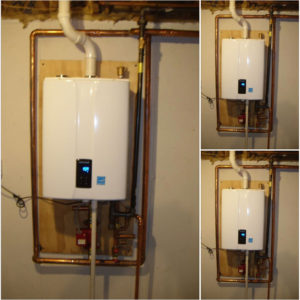This set of images depicts an indoor utility room featuring a tankless water heater mounted on a wooden board. The main unit, occupying the central focus of the photos, is white with a notable black display panel. This panel features an unreadable green light along with an illuminated blue logo or text. The image set includes one large photo on the left, taking up about two-thirds of the frame, and two smaller, identical photos on the right, each occupying half of the remaining space. The water heater is encased in a system of copper pipes and a PVC pipe that extends from the top of the heater into the ceiling, likely part of the unit's ventilation or exhaust system. A black power cable can be seen connected from the left of the heater, while additional copper piping runs from the bottom, correlating with its function of heating water. The surrounding environment acts as a backdrop, highlighting the intricate plumbing and electrical setup necessary for the water heater's operation.